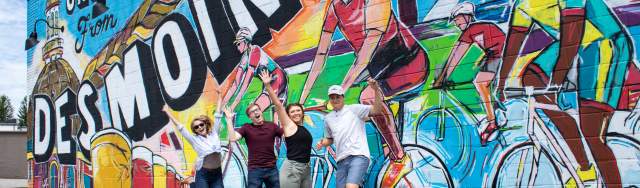The photograph captures a lively scene of four people—two men and two women—jumping and leaping in joy in front of a colorful graffiti mural in Des Moines, Iowa. The mural, in the style of an old-fashioned postcard, prominently displays bold white letters spelling "DES MOINES" but is partially cut off at the "I" and "N." The artwork depicts a cycling race with cyclists dressed in yellow, blue, and red outfits, and features a monument with a dome steeple and a streetlight. The sky above the mural includes the word "From."

In the foreground, the four individuals are mid-jump with their hands in the air, except for the man on the far right, who has his arm slightly raised. The woman on the left sports a white blouse, dark-colored pants, blonde hair, and sunglasses, revealing her midriff. Next to her is a man in a maroon shirt and dark jeans, mouth wide open in excitement. The woman next to him wears a black halter top and gray shorts, and the man on the far right dons a white baseball cap, a white shirt, and blue denim shorts. The exuberant expressions and animated poses of the group contrast vividly with the dynamic graffiti background, creating a spirited and celebratory atmosphere.